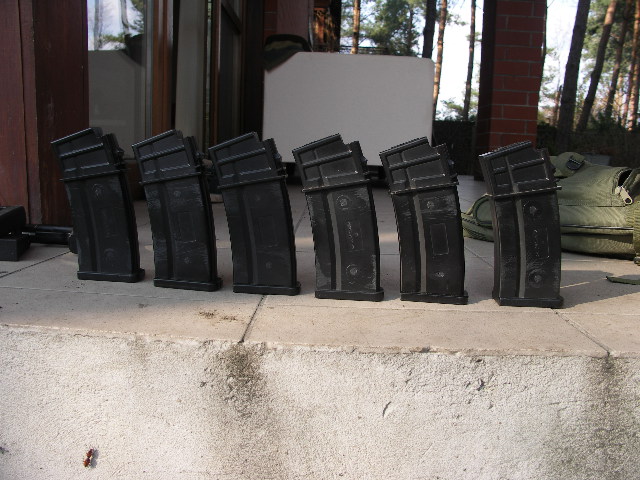In this color photograph taken outdoors, six black canisters, which might be vents or even resemble ammunition magazines, are sitting on a cement-tiled patio. Each canister is rectangular with a slight curve to the left, standing approximately 12 to 18 inches tall. Behind these figures is a large square black structure. The patio features raw cement edges topped with tiles. To the right of the canisters rests a green zippered pouch or backpack. From the patio, large tree trunks and green foliage are visible, along with a hint of light glimmering between the trees. Additionally, the background includes wooden doors with glass window panels, a red brick column, and what appears to be a folded plastic table. The left side of the image reveals parts of a building with greenish and brownish panels.